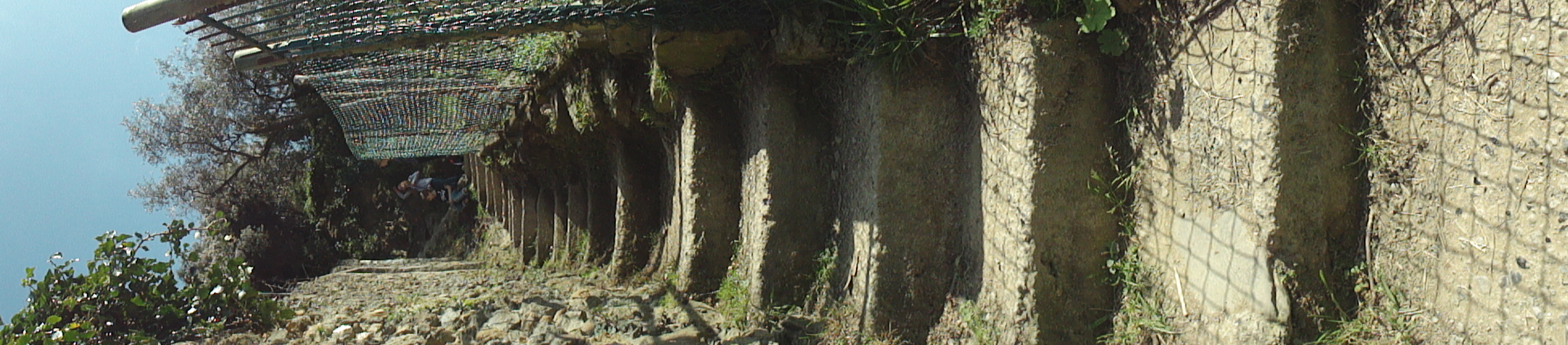In this panoramic photograph, the central focus is on a unique architectural structure on the right consisting of an ancient wall with repeating segments, each about half a foot before arching into another section. These wall segments, which appear to be eroded or overtaken by nature, give an impression akin to dominoes. The structure, which looks like it could be part of a lost temple, is made up of square tiles in gray and tan colors, some of which are outlined in what appears to be cement. Ivy and other greenery seem to be creeping up these walls, adding to the ancient, abandoned feel.

To the left of the walls, there is a peculiar canopy made of ropes and potentially stitched materials, resembling a hut ceiling or an improvised shade structure. Further left, the image reveals a light blue sky and more greenery, including trees hanging over the top of what appears to be a roof. 

The ground is covered in dirt with rolled-up lines suggesting some manual activity. Steps or a pathway lead downward through the structure, and in the backdrop, a group of people, possibly engaged in physical labor, is visible. They are dressed in tan hats and working in a space surrounded by greenery. This scene merges historical architecture and natural elements, capturing both the decay and the resilience of the landscape.